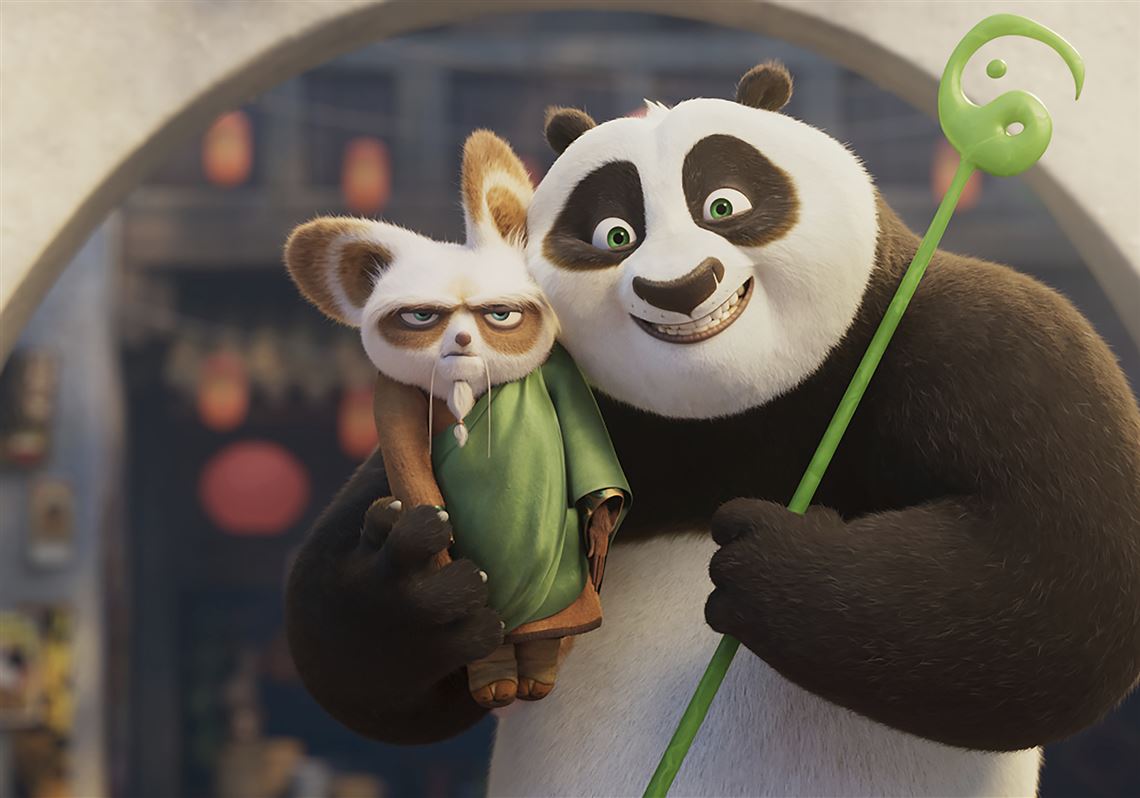This is a detailed color image featuring the cheerful panda from "Kung Fu Panda" standing to the right. The panda is smiling widely with an expression that glows from cheek to cheek, holding a distinctive light green scepter in his left hand. The scepter features a yin-yang symbol at the end. In his other arm, the panda is gently holding a small creature with a white face marked by brown circles around its eyes, a brown nose, large white and brown striped ears, and wearing a green, sideways-slung tunic resembling a monk’s attire. The small creature appears visibly annoyed, its mouth set in a straight, disgruntled line and a furrowed brow emphasizing its displeasure, arms stiffly hanging down by its sides. The background is a blurry mix of colors and details, with red lanterns and a prominent arch fading into tan at the upper left and right sides, ascending to form a brown arch overhead. This animated drawing vividly displays the contrasting expressions and personalities of the panda and his unwilling companion.